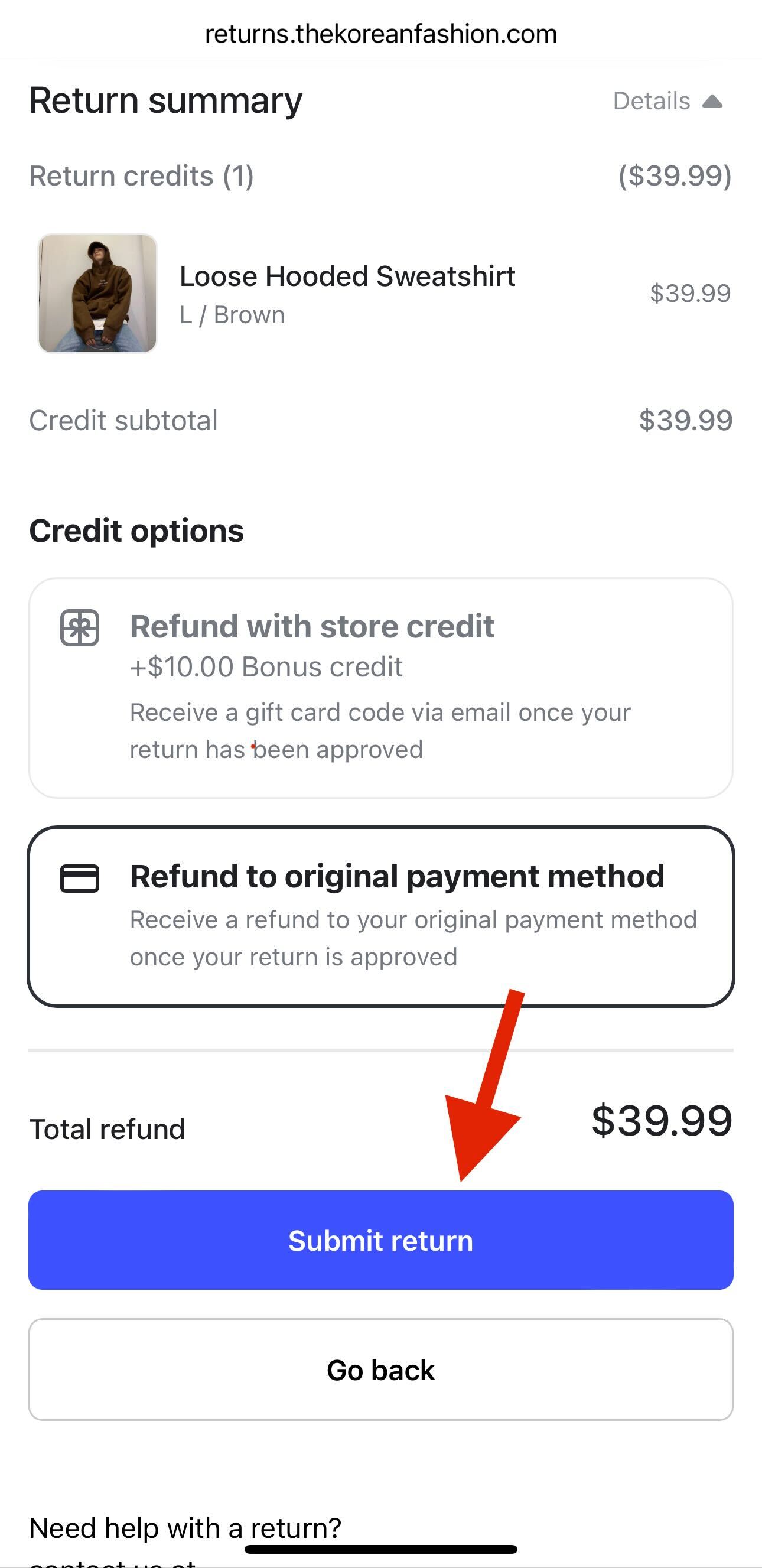The image for the shop is a vertical rectangle layout that begins with the URL "returns.thekoreanfashion.com" at the top. Below, the section titled "Return Summary" is prominently displayed in dark black text. On the right-hand side of this section, there is an option labeled "Details" with an upwards arrow.

Underneath the "Return Summary," a line indicates "Returns Credit" followed by the number 1 in parentheses, accompanied by the amount ($39.99) also in parentheses. The next line features an image displaying a person wearing a loose hooded sweatshirt, with "Loose Hooded Sweatshirt" written in bold print. Below the product name, the size and color "L / Brown" are indicated in lighter print. Adjacent to this description, in the right column, the price "$39.99" is noted.

Following a white space, the "Credit Total" of $39.99 is mentioned in gray text. Moving on, the section "Credit Options" is presented in darker black text. Within this section, there are multiple options listed:

1. "Refund with store credit," accompanied by a note for an additional "$10 bonus credit."
2. "Receive a gift card code via email once your return has been approved."

The selected option in this image is "Refund to original payment method," described further as "Receive a refund to your original payment method once your return is approved." 

Finally, the "Total Refund" amount of $39.99 is indicated alongside a red arrow pointing downward towards a blue box labeled "Submit Return," and another box that says "Go Back."